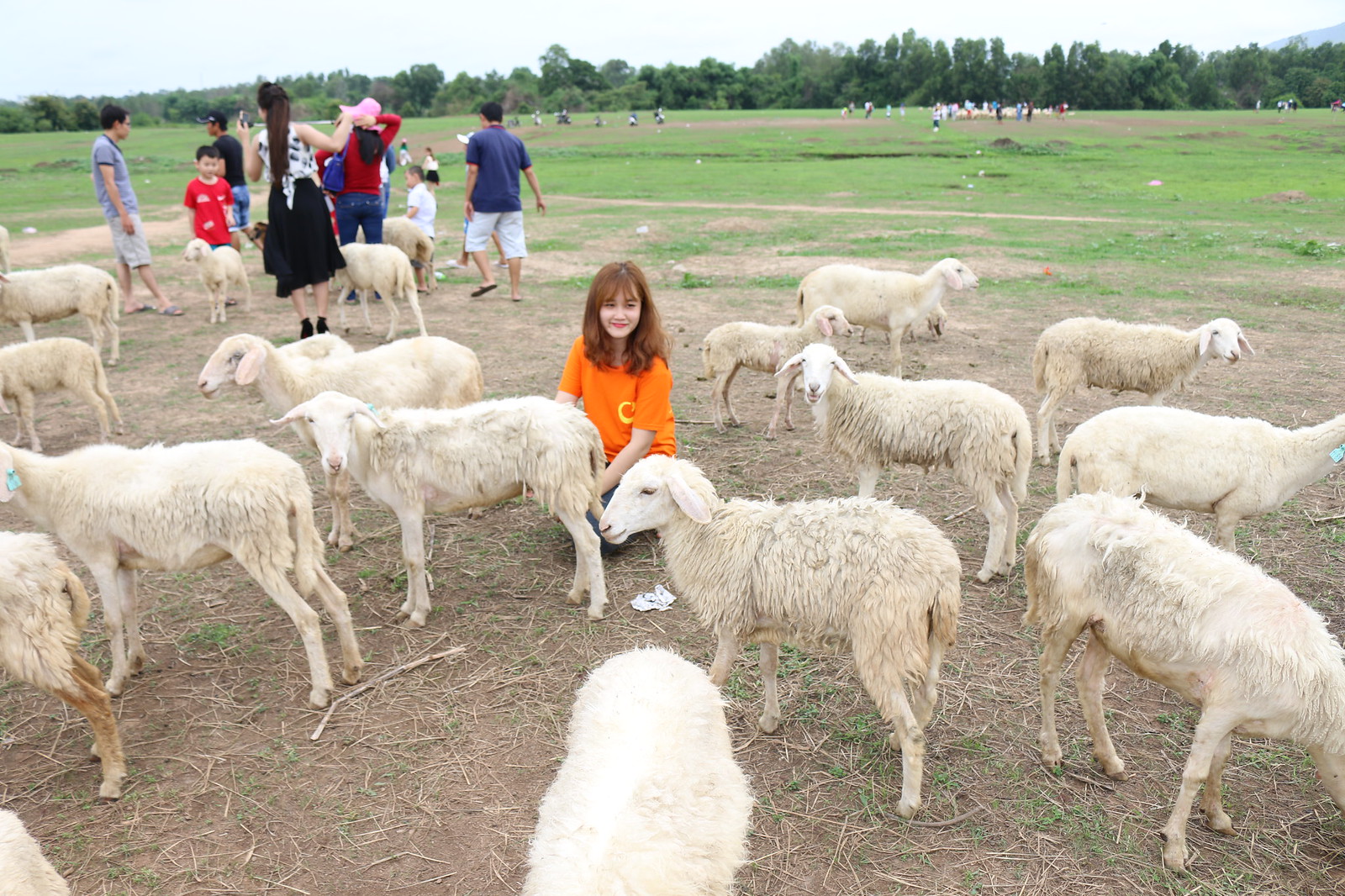The photograph captures an outdoor scene dominated by a group of approximately 15 white and light-gray goats scattered across a straw and dirt-covered ground. Central to the image is a young woman with shoulder-length reddish-brown hair, wearing a bright orange T-shirt with a yellow logo and jeans. She is on her knees, smiling gently as she looks at one of the goats. In the background, to the left, stands a mixed group of seven people, including men, women, and a child in a red shirt, engaging with the goats. The scene transitions into a green pasture that ends at a line of lush, varying-height trees. The horizon features an overcast and dusty-looking sky, giving the overall scene a rustic, pastoral feel.